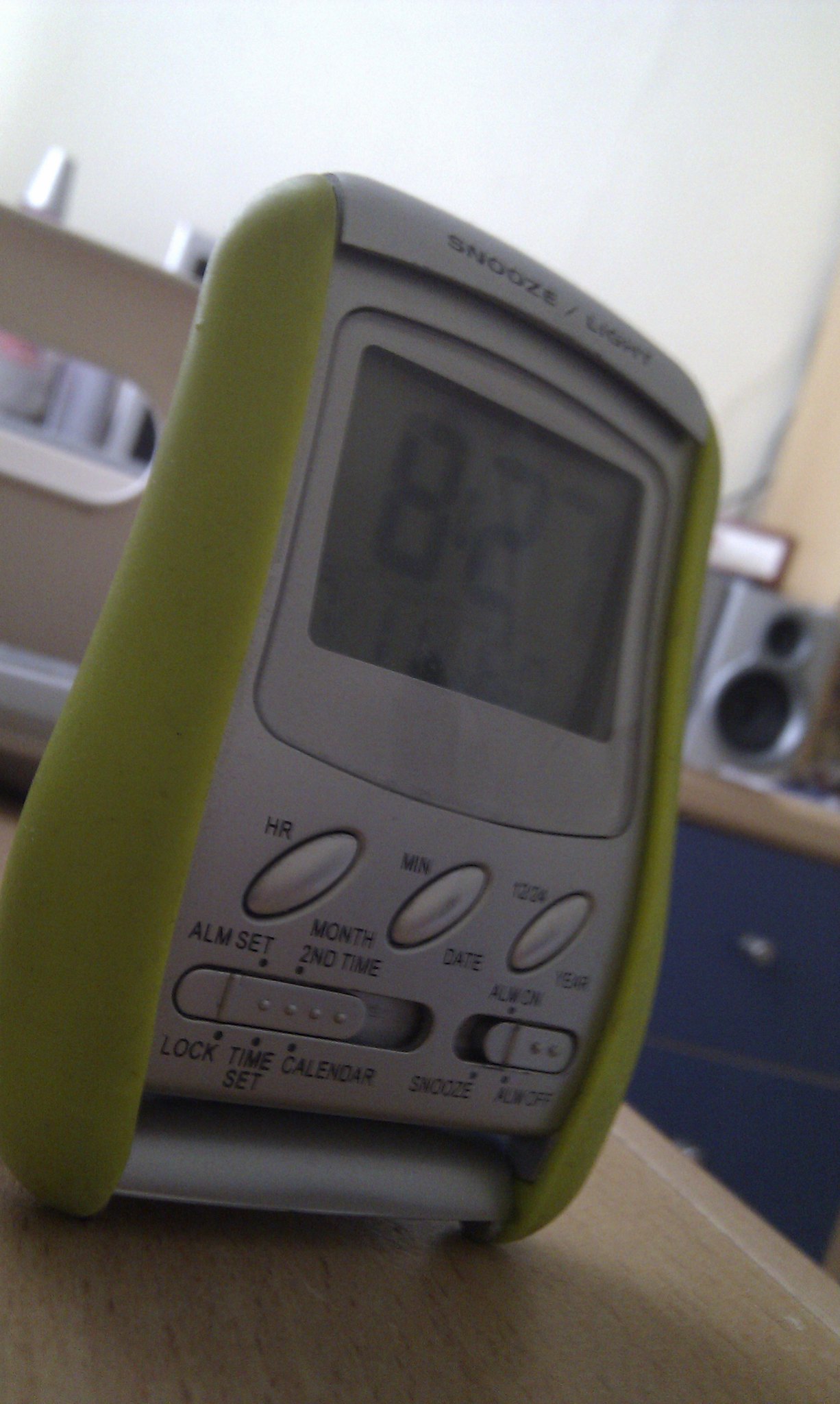In this image, a rectangular digital clock is prominently displayed on a wooden table in the foreground. The clock features light lime green sides with a silver-toned center that has black text. Its white face displays the time 8:27. Above the clock face, "Snooze/Light" is clearly marked. Below, several buttons are visible, labeled for various functions including "Hour," "Minute," "Alarm Set," "Month," "Second Time," "Date," "Year," "Lock Time," "Calendar Set," and "Snooze." In the background, there are small pieces of furniture, providing additional context to the setting.